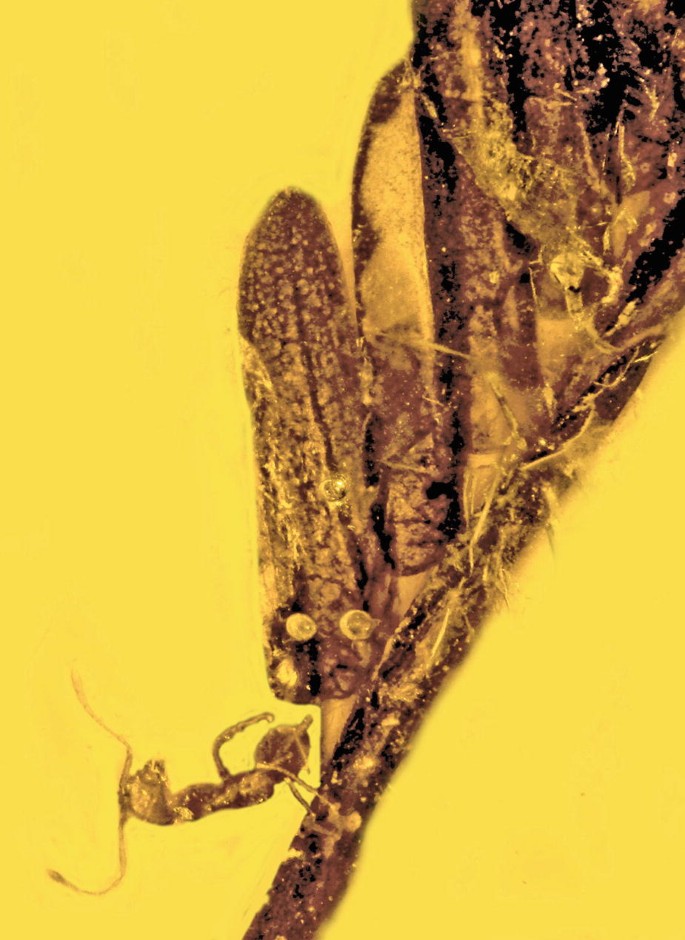This detailed image captures a fossilized scene within amber, showcasing a brown, distorted ant standing on a long twig, with its body twisted around, possibly due to the sap's movement or hardening process. The overall color palette of the photo features various shades of brown, dark yellow, and the glowing yellow hue of the amber itself. Surrounding the twig are several oblong shapes, which might be leaves or seed pods, giving the impression of an ancient, encapsulated environment. The ant appears to be precariously balanced, touching the twig with only its two rear feet, further adding to the image's intricate details. The leaf it stands on seems dried and fibrous, contributing to the rustic texture and depth of the scene.